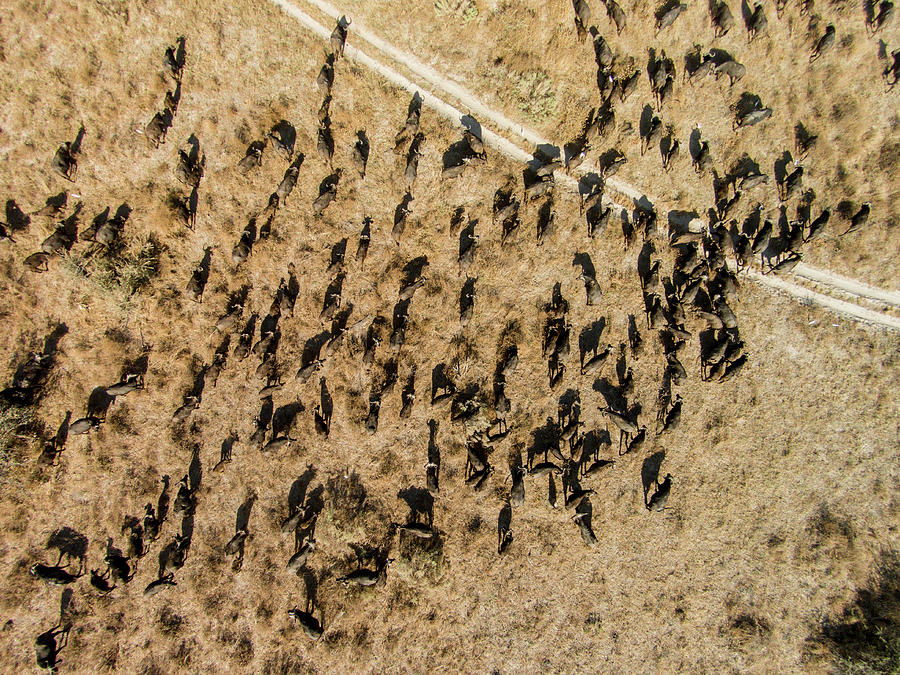This aerial photograph captures a sprawling field of dry, yellow grass, segmented by an old dirt road running through the middle. The expansive landscape is populated by a large herd of dark-colored, likely black cattle, scattered uniformly across the grassland. Some of the cattle cluster tightly together, while others are more spread out. The shadows cast by the animals reveal antlers or horns, adding to the intriguing detail of the image. On the lower right side, there is a noticeable drop-off, suggesting a hazardous area where any animal could get seriously hurt if they fell. The vantage point, likely from a drone or a low-flying plane, provides a bird's-eye view of this fascinating and dynamic scene, capturing the essence of a large herd navigating through a parched, yet picturesque landscape.